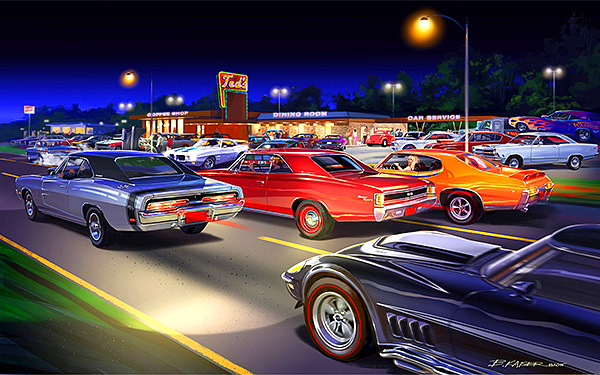The image portrays a richly detailed, computer-generated night scene reminiscent of the 1960s or early 70s, featuring a collection of vibrant and classic muscle cars around an establishment named Ted's. The establishment, adorned with neon signage, serves as both a dining room and a car service, embodying the style of vintage drive-ins. The dark, deep-blue sky is punctuated by glowing streetlights that give the scene an atmospheric glow, enhancing the vivid orange, red, gray, purple, and blue hues of the cars. The street, marked by clean yellow lines, hosts several lanes of traffic with cars driving or parked around Ted's. Notable cars include a Corvette Stingray, old Chevrolets, a Chevelle, and a hot rod with a distinctive rainbow fire detailing. The parking lot is busy, with cars' headlights illuminating the area. Ted's itself has a brightly lit sign in orange and red, advertising both dining and car service, hinting at an inviting blend of nostalgia and vibrant nightlife. The scene captures a moment frozen in time, evoking the spirited culture of classic American car shows and diners.